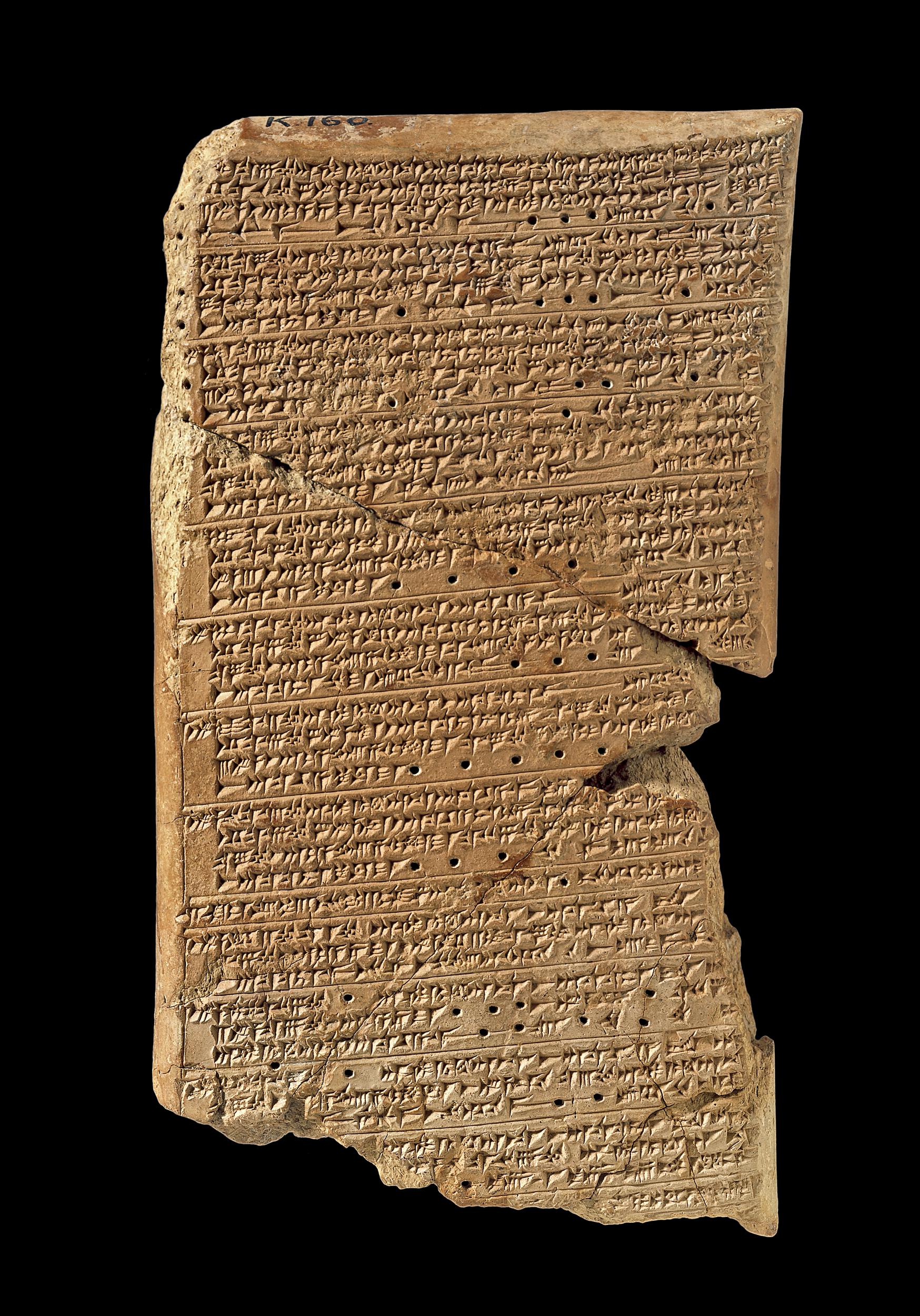This photograph features an ancient tablet displayed against a stark black background, likely in a controlled environment such as a museum. The tablet is sandy beige in color and made of what appears to be a sandstone material. It bears intricate engravings of ancient text or hieroglyphics divided into twelve distinct sections by horizontal lines. The writing does not correspond to any known modern language, and its exact origins and meaning remain uncertain.

The tablet itself is roughly rectangular in shape, but its edges are uneven and not uniformly smooth. The top, right, and left edges appear relatively intact, while the bottom edge is notably broken into irregular chunks, giving the piece an incomplete appearance. Additionally, the right side, particularly towards the bottom, exhibits multiple chips and missing fragments.

Significantly, the tablet has been fractured into three main parts. One crack runs diagonally across the top third of the tablet, while another fissure traverses the lower section, creating a distinct triangular middle piece whose apex is slightly rounded. Despite these breaks, the pieces have been carefully repositioned to join together and present a coherent view of the artifact's engraved text, underscoring the artifact's historical and cultural significance.